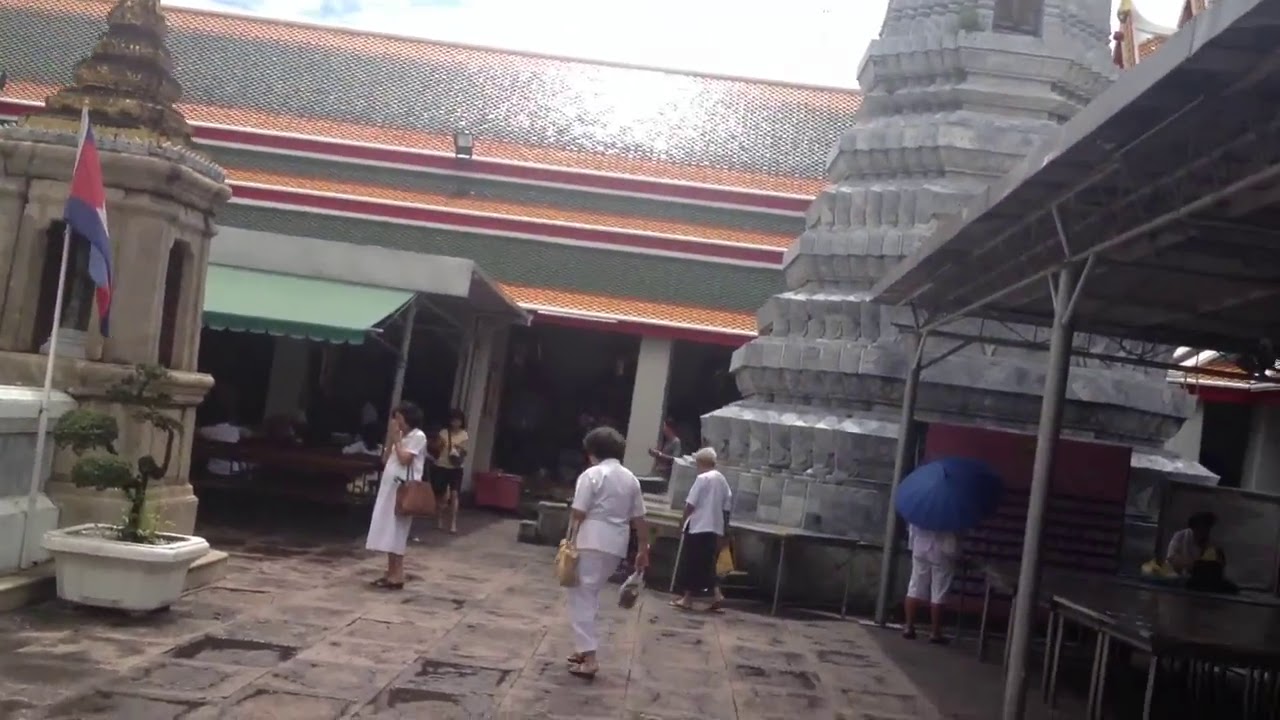The image depicts a bustling marketplace in an Asian country, characterized by a blend of traditional and modern elements. The centerpiece is a vibrant outdoor square where several elderly women, dressed in white, traverse the area carrying yellow and other colored bags. The ground is paved with rough brown tiles, some showing darker patches or possibly puddles. Dominating the image is a large, multi-colored tiled roof, with orange, green, and red stripes, angled prominently from the top left. 

To the right, a large, cone-shaped gray concrete column stands, while on the left, there is a layered traditional tower, possibly a sculpture, and a white flagpole bearing a red, blue, and white flag. Nearby is a potted plant containing a small bonsai tree. Canopies shield the market stalls, with a green canopy visible to the left. Adding to the scene, a person clad in white holds a blue umbrella on the right side of the image. The colorful roof, traditional objects, and the mix of people and merchandise convey the rich cultural tapestry and daily life in this Asian marketplace.